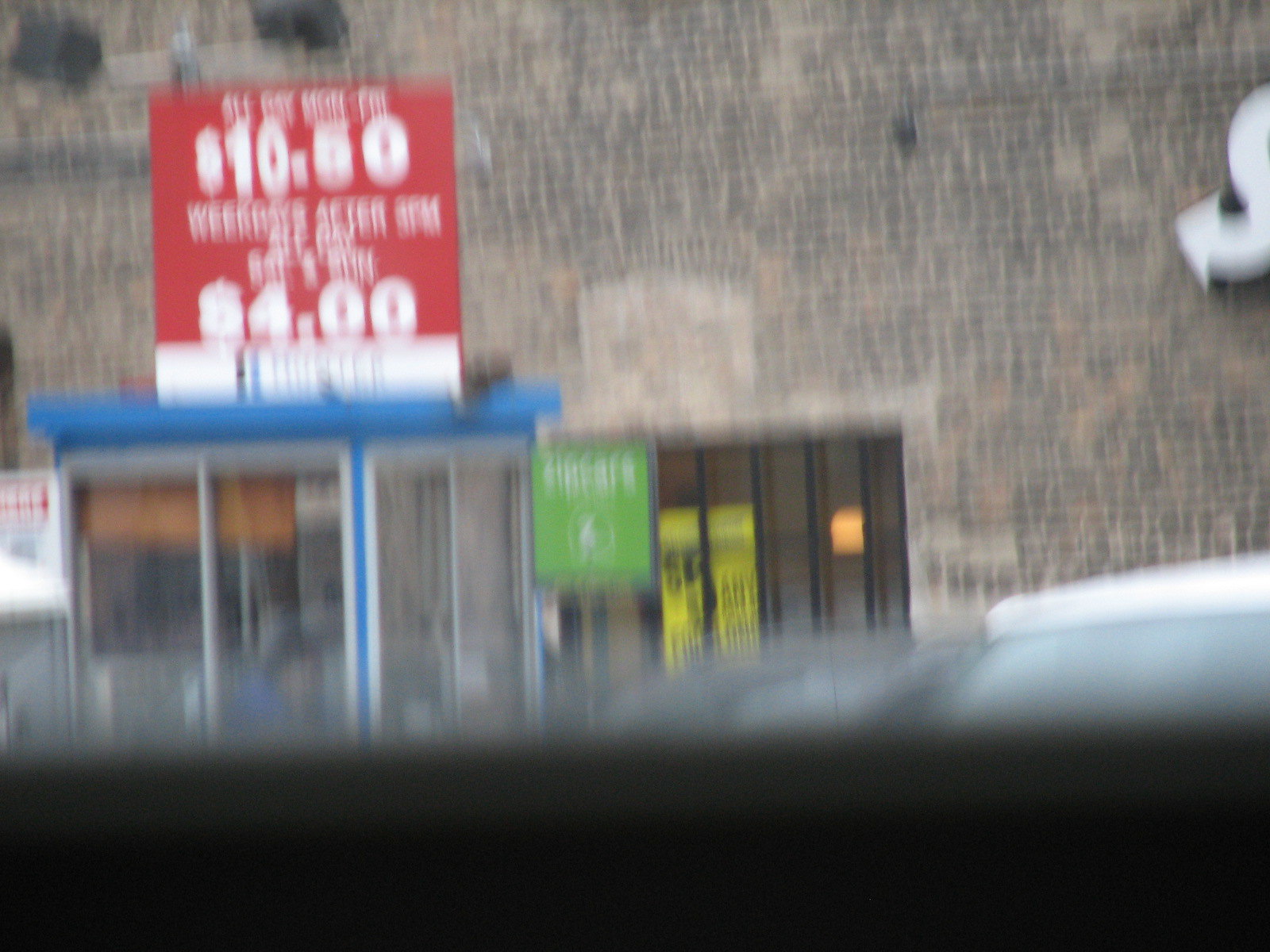This image is a very faded and blurry photograph, possibly taken from inside a car due to the appearance of a ledge in the frame. The primary focus is a small, rectangular building which might function as an office or a small store. The building is characterized by a blue roof, and its front facade is predominantly glass, giving it a modern, transparent appearance. 

Above the building, there is a red sign or billboard with white lettering, partially readable, displaying "$10.50" and "$4," with some unreadable text between these numbers. Additionally, there are two distinct signs on the building: a green one centrally placed and a yellow one as well. The building's structure and signs suggest a commercial establishment, possibly a small service outlet or retail space. The overall setting hints that the building might be situated in a public or semi-public space, potentially near a bus stop or a busy area frequented by pedestrians.